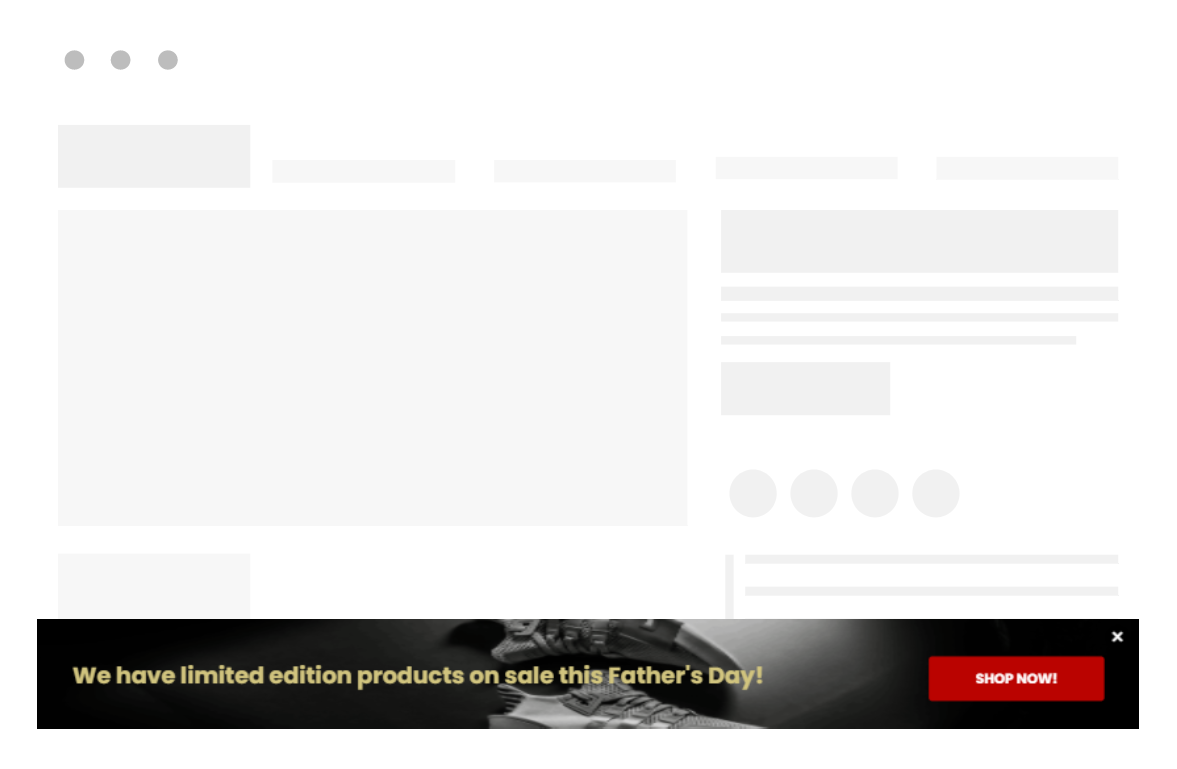This image showcases a website screenshot with most sections obscured except the bottom banner, which appears designed to demonstrate the placement and appearance of advertising banners. The prominently featured banner spans the bottom of the image, displaying a black-and-white advertisement for limited edition products on sale for Father's Day. Centrally positioned on the banner is a monochromatic image of a tennis shoe. To the right of the advertisement text, there's a rectangular red "Shop Now" button. Additionally, there is a small 'X' icon in the top right corner of the banner, suggesting the option to close the ad. The rest of the website's layout includes placeholder shapes: a large gray square and several smaller gray squares with a series of gray circles on top, likely indicating where future content or website elements will be placed.